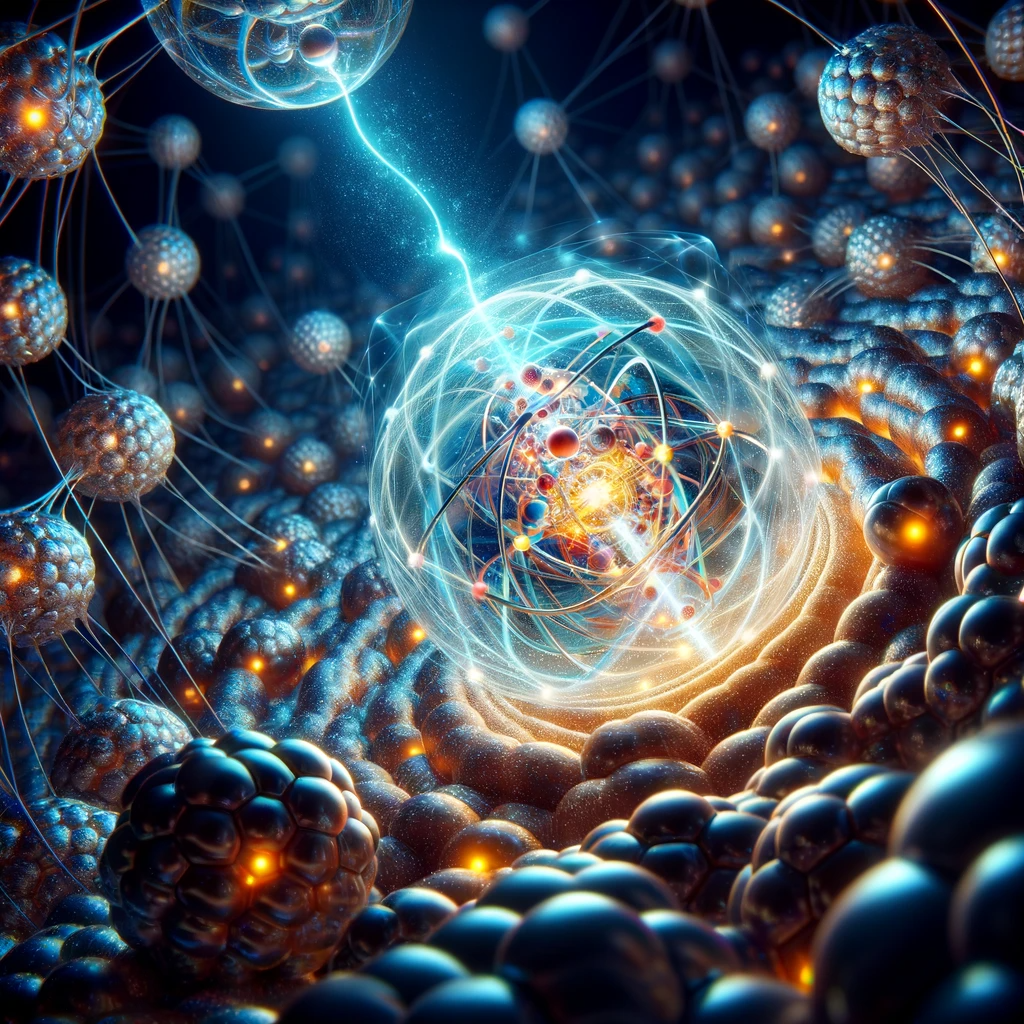This digital illustration is a highly detailed, sci-fi inspired depiction of a microscopic world at an atomic or molecular level. Central to the image is a spherical "timepiece," emitting a radiant orange and yellow light, encircled by a vortex of energy beams. Surrounding this core are numerous interconnected, globular structures that appear almost like dark blue or grayish-black berries, complete with a bumpy texture resembling raspberries or blueberries. These orbs are linked together by delicate, thread-like filaments, creating a web-like network. Many of these globular spheres contain a glowing orange or yellow spot at their cores, adding to the intricate display of light and energy. The entire composition is bathed in an array of blue, silver, and gold hues, with white and aqua energy beams threading throughout the scene, lending a dynamic, electrified atmosphere to the artwork. The detailed interplay between the interconnected orbs and the vibrant central sphere gives the illustration a sense of both complexity and depth, capturing the essence of a fantastical, microscopic universe.